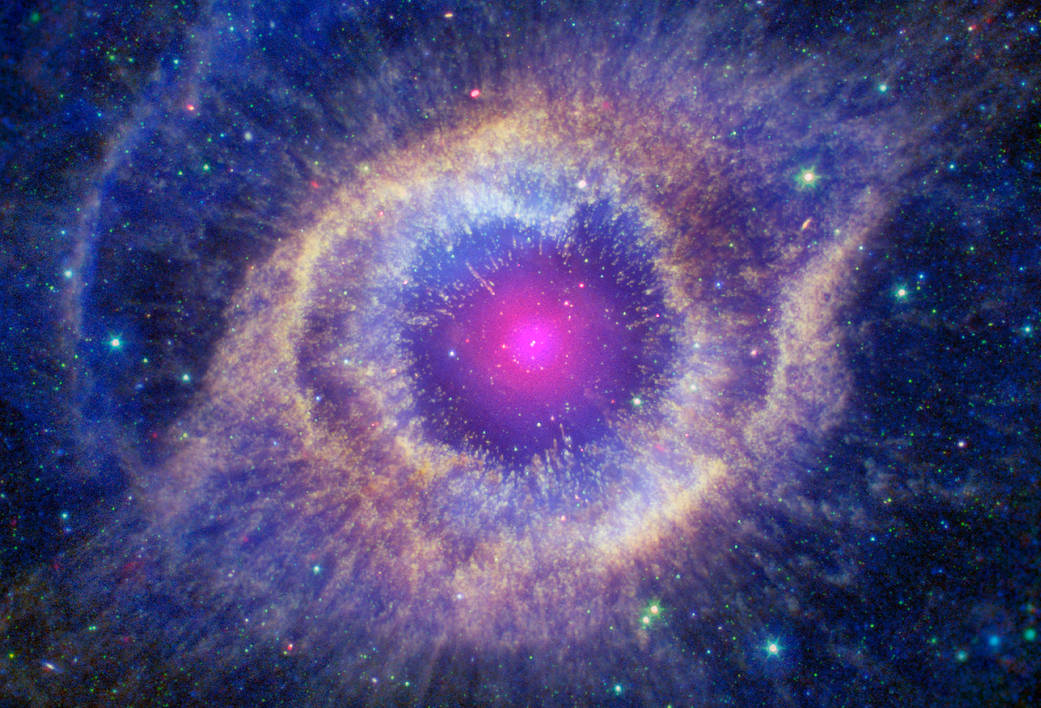The image captures a mesmerizing telescope view of a nebula, set against a dark navy blue background speckled with an array of stars in varying sizes and intensities. Dominating the frame are gaseous rings arranged in a pattern of concentric circles, displaying a rich palette of colors. At the heart of the nebula, a glowing, blurry circle in shades of violet and reddish-purple creates a vibrant focal point. The gas thins out in this central area, allowing the starry field to become more pronounced. Surrounding this core are rings of varying hues, beginning with darker patches, then transitioning into bright yellow and orange rings. Further out, a thin bluish ring blends with the stellar speckled background, interspersed with points of light in pink, green, and white. This celestial display culminates in the faint, yet vivid, outer edges of the nebula, creating a magnificent spectacle of color and light against the vast expanse of space.